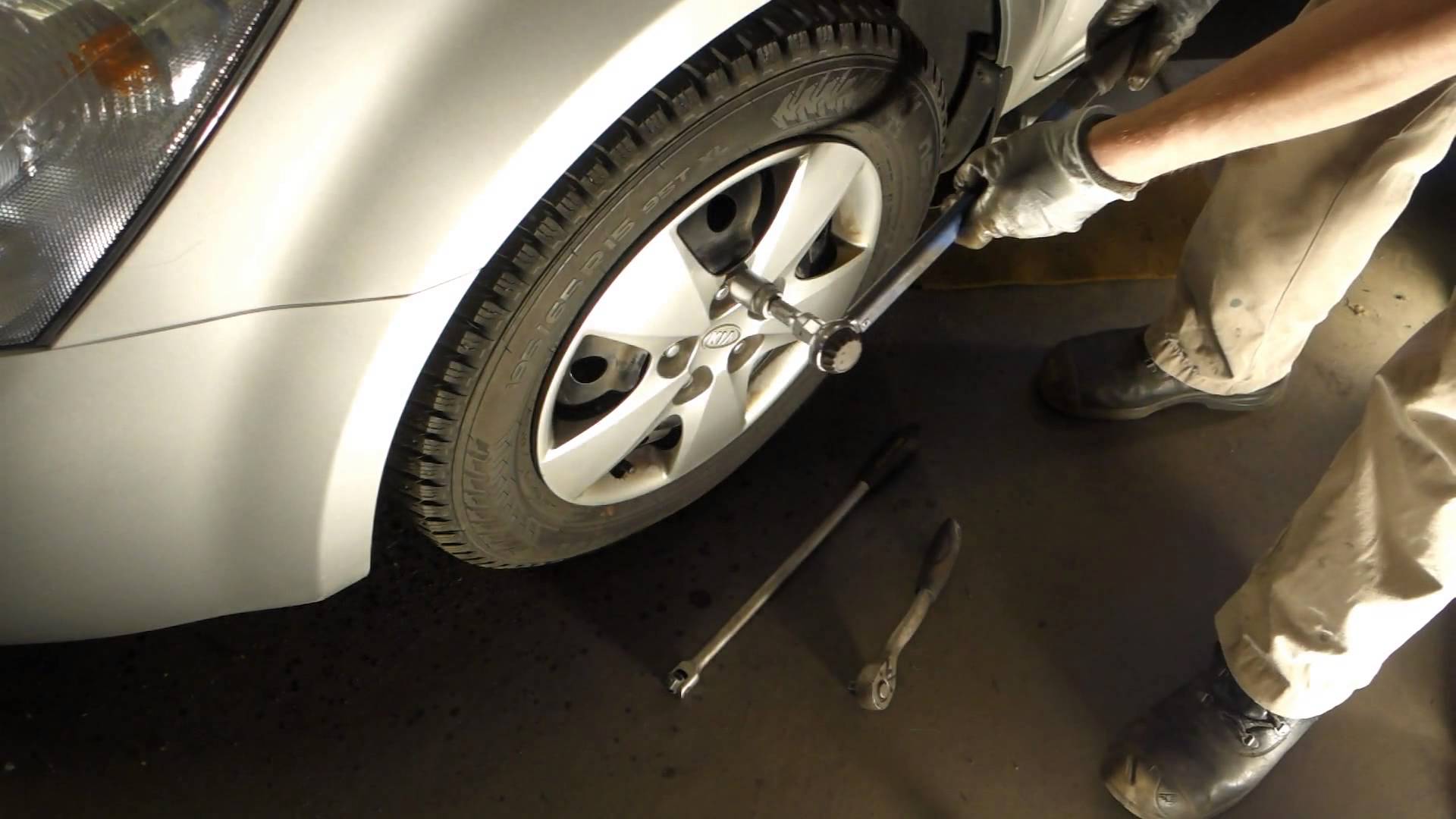The photograph is a close-up shot of the driver's side of a grayish silver Kia vehicle, potentially a sedan or SUV. The image focuses primarily on the driver’s side tire, which prominently displays the brand name "Kia" and tire measurements. The partial headlight and a sliver of the front bumper can also be seen.

In the foreground, a person is working on the tire. Visible from the knees down, the individual is dressed in long tan pants, black lace-up shoes, and gloves. The left arm, visible from the elbow onward, is bare except for the glove, while only the fingers of the right hand are visible, suggesting a sleeve is covering the rest of the arm. The person is using a tool attached to the tire rim, presumably performing maintenance or repairs. Two additional tools lie on the ground near the worker. The image captures a moment of focused manual labor, highlighting both the vehicle and the tools used in its upkeep.